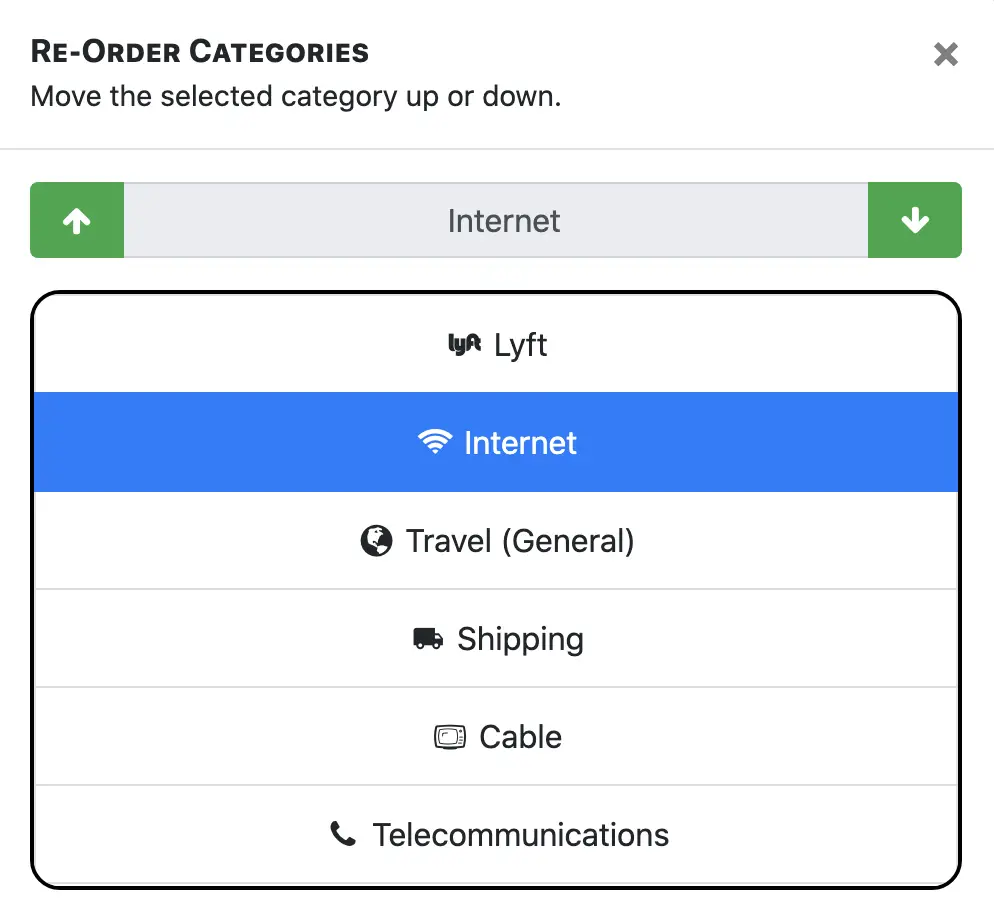This is a screenshot depicting a menu within an app, featuring a white background. At the top-left corner, the title is displayed in bold black font: "Reorder Categories," followed underneath in standard font with the instruction: "Move the selected category up and down." Adjacent to this text on the right is a small gray 'x.' Directly below this is a faint horizontal line in black, followed by a gray rectangle. 

Within the rectangle, on the left end, there is a green square with a white arrow pointing upwards, and on the right end, a similar green square with a white arrow pointing downwards. Centered between these arrows is the word "Internet." Beneath this, there is a black-outlined square containing a list of options in white rectangles, each labeled in black font.

The options, ordered from top to bottom, are as follows:
1. "Lift" – accompanied by the Lift symbol to its left.
2. "Internet" – accompanied by a Wi-Fi symbol.
3. "Travel (General)"
4. "Shipping"
5. "Cable"
6. "Telecommunications"

Each item in this list is prefixed with a small icon relevant to its category, enhancing the visual guide for users navigating the menu.